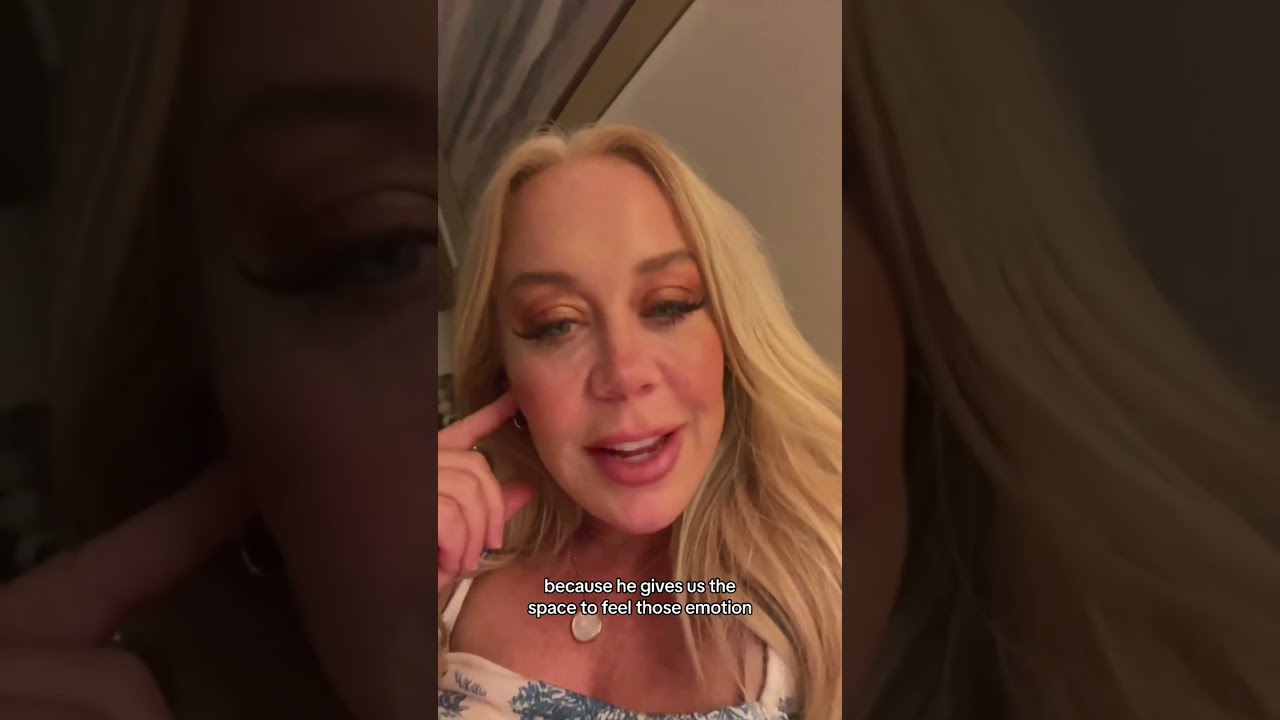The image features a middle-aged, blonde-haired woman with long hair cascading over her shoulders. Her roots are brown, and she is adorned with striking makeup, including vibrant pinkish eye shadow, heavy rouge on her cheeks, and dark mascara-coated eyelashes. Her right eye appears slightly less open than her left. She wears dark lipstick that accentuates her prominent lips, and has a partially open mouth showcasing her white teeth, suggesting she might be speaking. Her hand is raised to her face, with her index finger pointed towards her ear and thumb towards her cheek, while her other fingers form a loose fist. She is dressed in a white garment with a low neckline that features blue floral patterns, possibly a tank top or dress, though the exact length is unclear. Around her neck, she has a delicate necklace with a silver or golden pendant. The central rectangular image of the woman is superimposed onto a larger, darker, and highly magnified background of her own face. This creates an effect where portions of her head appear to be split and expanded behind the main portrait. The backdrop includes a tan wall and a brown curtain. Beneath her face, there's a white text overlay that reads, "because he gives us the space to feel those emotions."